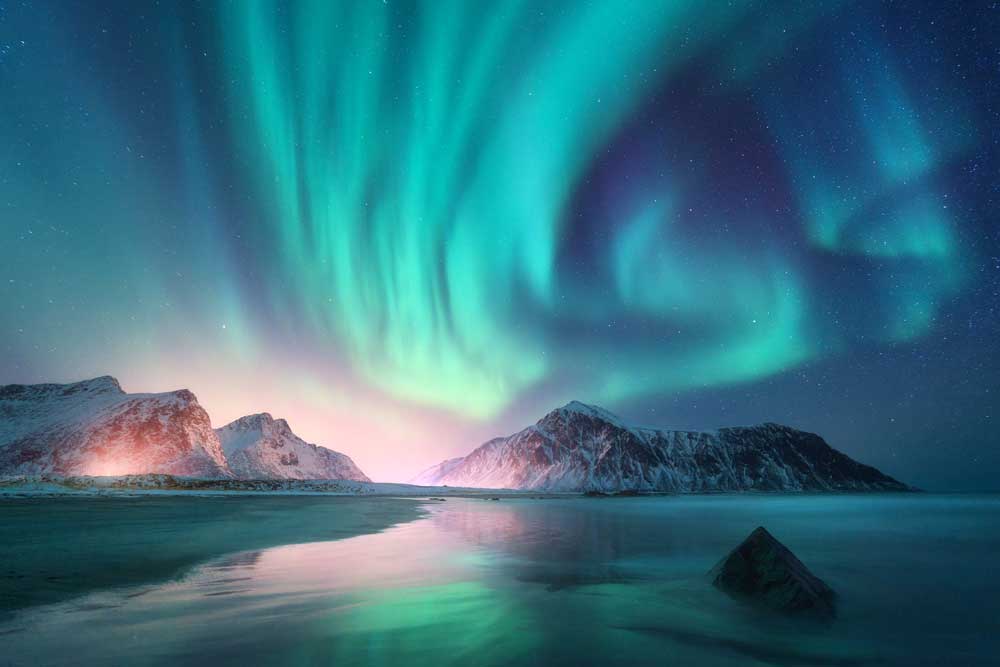The image portrays a breathtaking and cold nighttime scene featuring the Aurora Borealis. Above, a star-filled sky is illuminated by swirling, vibrant light phenomena in shades of green, light blue, and light purple—the auroras. The scene is set on the water, which mirrors the enchanting colors of the northern lights. In the distance, snow-covered, rocky mountain peaks frame the grandeur of the aurora, with one mountain to the right and another to the left, creating a natural gateway through which the lights seem to emerge. The water below is partially frozen, with a small rocky point poking out in the foreground, enhancing the wintry atmosphere. Reflecting the auroras, the lake's surface ranges in hues from dark to shadowy blue, creating a serene yet striking contrast to the dancing lights above.